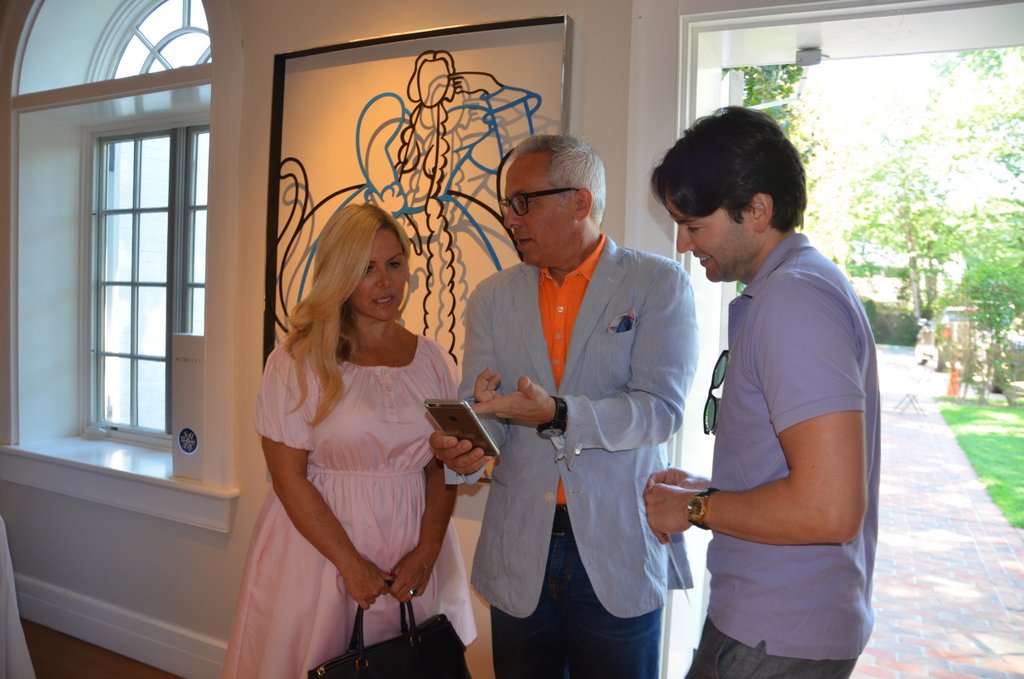This image captures the interior of a building, possibly a house or a church, with an open doorway leading outside to a sidewalk and grassy area. Dominating the scene are three individuals focused on a cell phone held by the older man in the middle. The woman to his right sports a light pink dress, a black purse held at her waist, and long blonde hair with dark roots. The middle-aged man, approximately 60 years old, is dressed in a notable light gray suit jacket, an unusually bright orange button-down shirt, and blue jeans, complemented by black glasses and a black watch. He points to something on his Apple smartphone, which the woman also looks at attentively. To his left stands a younger man in a purple polo shirt with sunglasses tucked into the neck, paired with gray shorts or pants. Behind them, the well-maintained wall hosts an almost abstract painting of a female figure in a poofy dress, depicted in a style resembling marker. The scene is imbued with a sense of activity and interaction, as if taking place at an open house or gallery event, further suggested by the open doorway facilitating easy access.